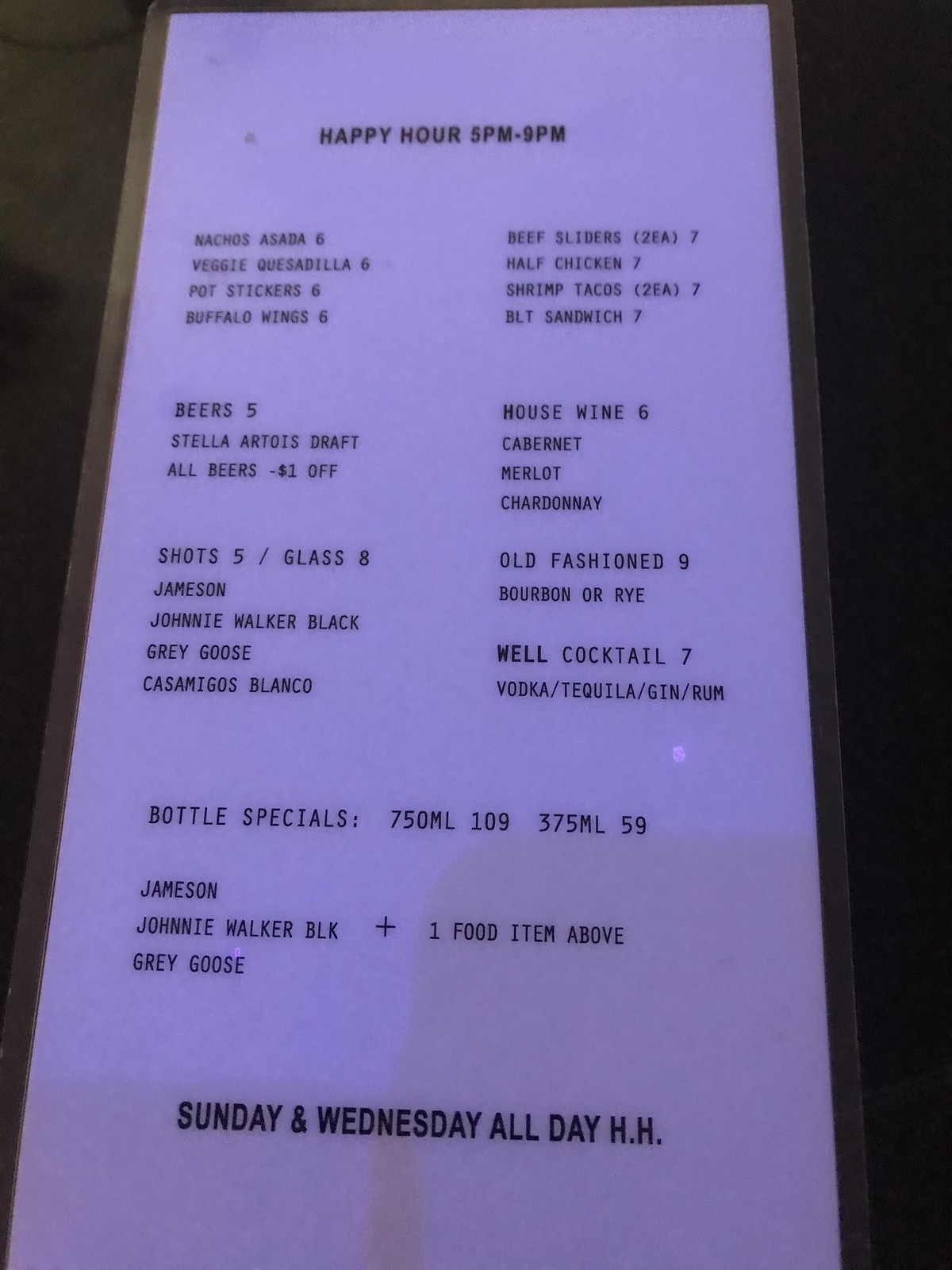The image captures a white, laminated happy hour appetizer menu, devoid of any logos or restaurant identifiers. At the top, it announces "Happy Hour 5-9 p.m." The menu presents a selection of eight appetizers, including nachos, asadas, veggie quesadillas, pot stickers, buffalo wings, beef sliders, and chicken and shrimp tacos, divided into $6 and $7 columns. 

The drink section lists beer options priced at $5, specifically mentioning Stella Artois and other beers for a dollar off. The house wine selection includes six varieties: Cabernet, Merlot, Chardonnay, among others. There's also a range of shots for $5 each, with premium options like Jameson, Johnny Walker Black, Grey Goose, and Casamigos Blanco available for $8 a glass. Classic cocktails such as an Old-Fashioned, available with either bourbon or rye, are priced at $9, while well cocktails are listed for $7. Additionally, there are bottle specials on Jameson, Johnny Walker Black, and Grey Goose. The menu highlights that happy hour is available all day on Sundays and Wednesdays.